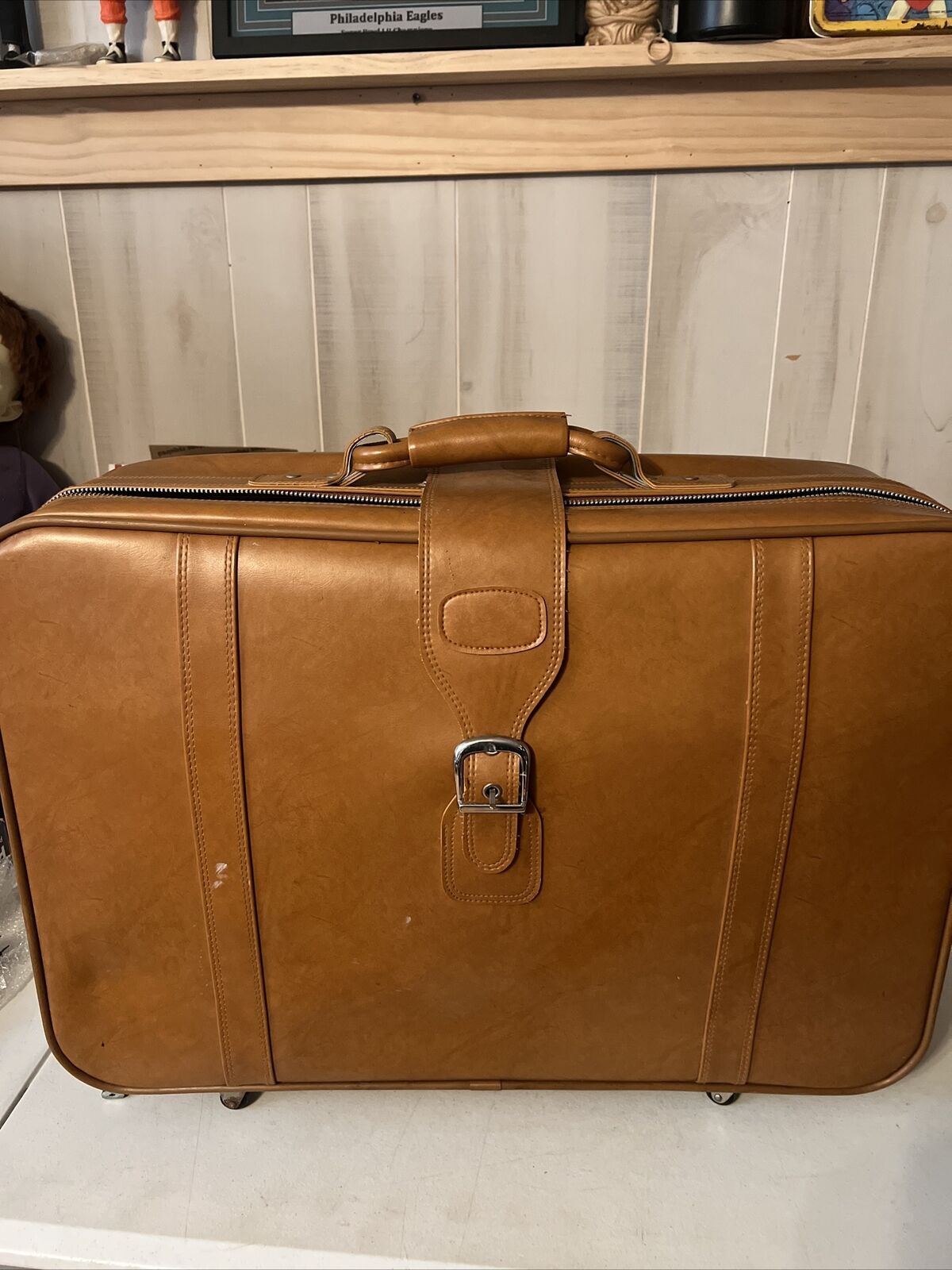This vertical photo features a vintage, camel-colored leather suitcase prominently positioned against a white paneled backdrop. The suitcase, devoid of wheels, has a classic design with a zipper that runs around it and a wide strap that secures with a buckle. It is equipped with a sturdy leather handle on the top. The floor beneath it is white, and behind the suitcase is a countertop, likely part of a well-lit room interior. The backdrop also includes an arrangement of vertical rectangular sections of varying sizes and a Philadelphia Eagles sign. Various objects are subtly visible, such as a figurine and some arts and crafts materials, lending a personal touch to the setting. The overall scene suggests someone might be preparing for a trip.